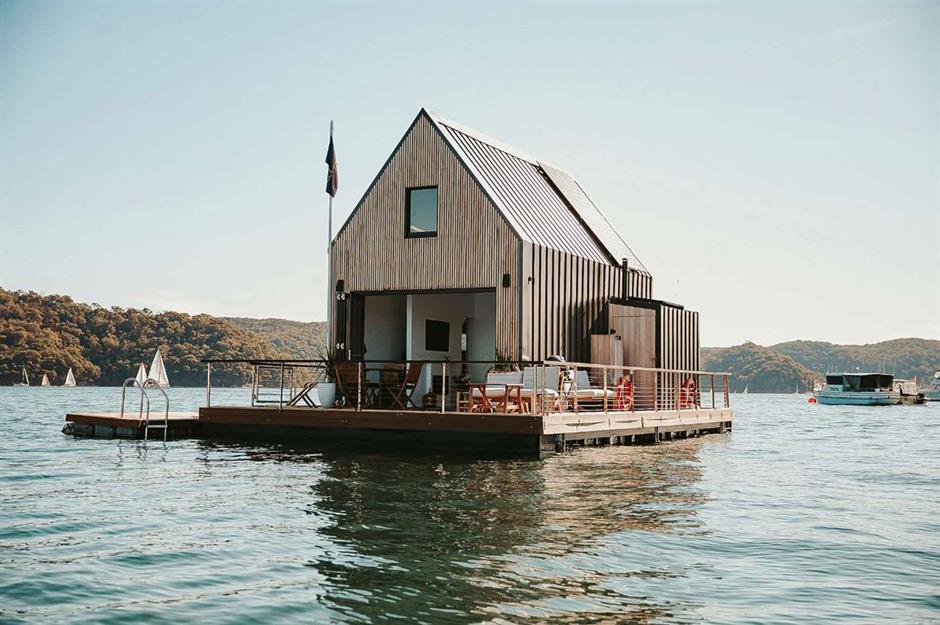The image captures a serene landscape featuring a unique floating wooden house, anchored on a square platform in the middle of a clear, calm lake. The barn-shaped house, tan in color with a single central window and a U.S. flag hoisted on a flagpole, is surrounded by an outer railing and adorned with various pieces of furniture both inside and outside. The platform also includes a small dock with a ladder on its left side, inviting one to climb up from the water. Around the house, the lake vividly reflects the structure, with sunlight glinting off the blue surface on either side and a warmer brownish tint in the center, mirrored from the house's color. In the background, additional similar platforms can be seen, along with several sailboats dotting the water. The lake is encircled by lush trees and rolling hills, leading to a harmonious blend of nature with the sky above transitioning into a soft yellowish-blue-gray hue. The right-hand side of the image shows a larger boat appearing on the horizon, enhancing the scenic beauty of this tranquil waterborne retreat.